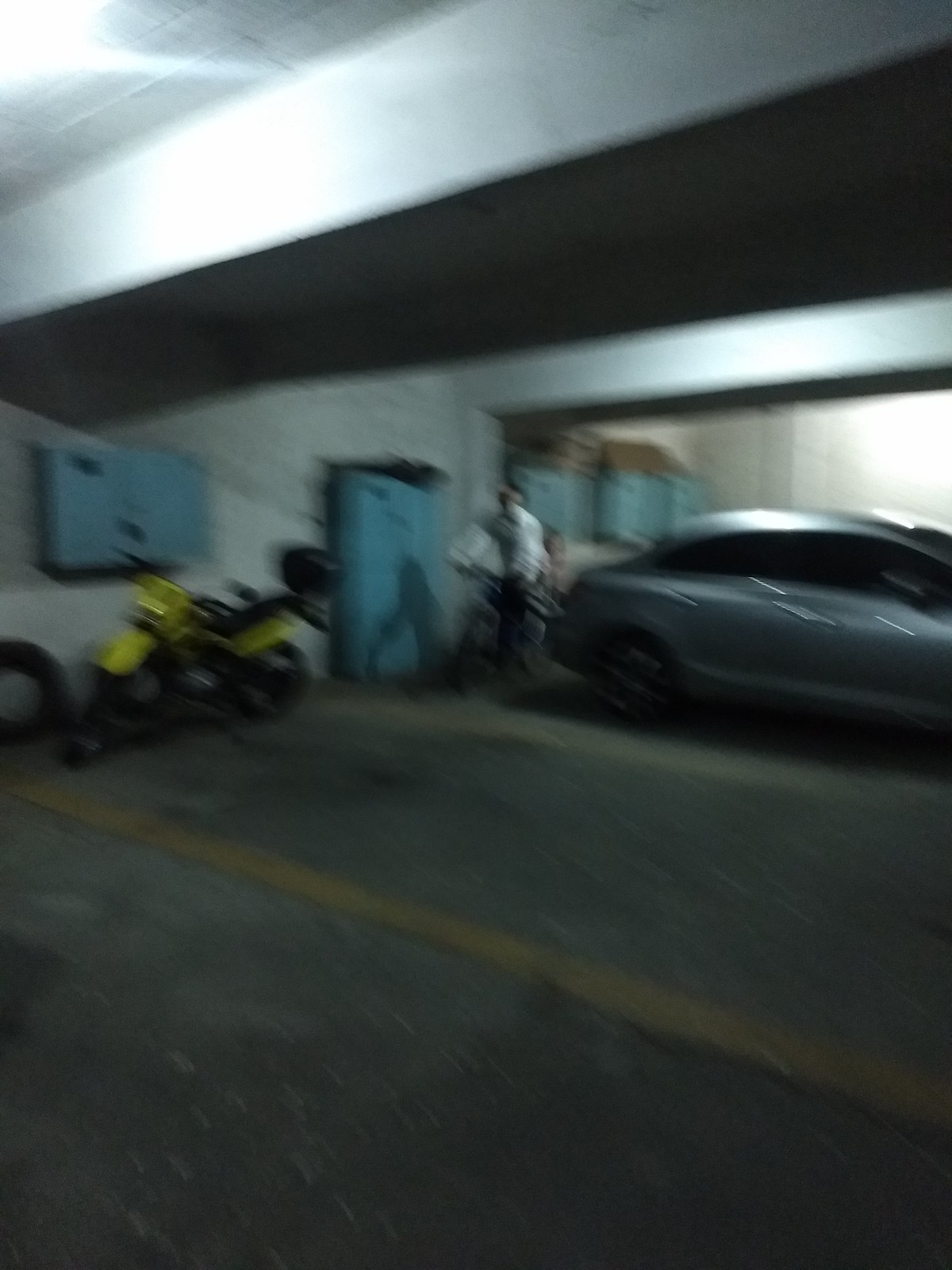The color photograph depicts a blurry, underground parking garage with low ceilings, concrete floors, and potentially stone or brick walls. Yellow parking lines designate the parking spots. In one spot near the end, a yellow motorcycle is parked sideways next to the wall, behind which blue utility cabinets are mounted. A man in a white shirt and blue pants, possibly on a bicycle or scooter, is seen in motion near a larger blue cabinet attached to the same wall. To the right of this man is a large silver car, and behind it, in another parking spot, is a second vehicle. Scattered throughout the background, more blue shelving units and a large concrete beam are visible, supporting the structure.